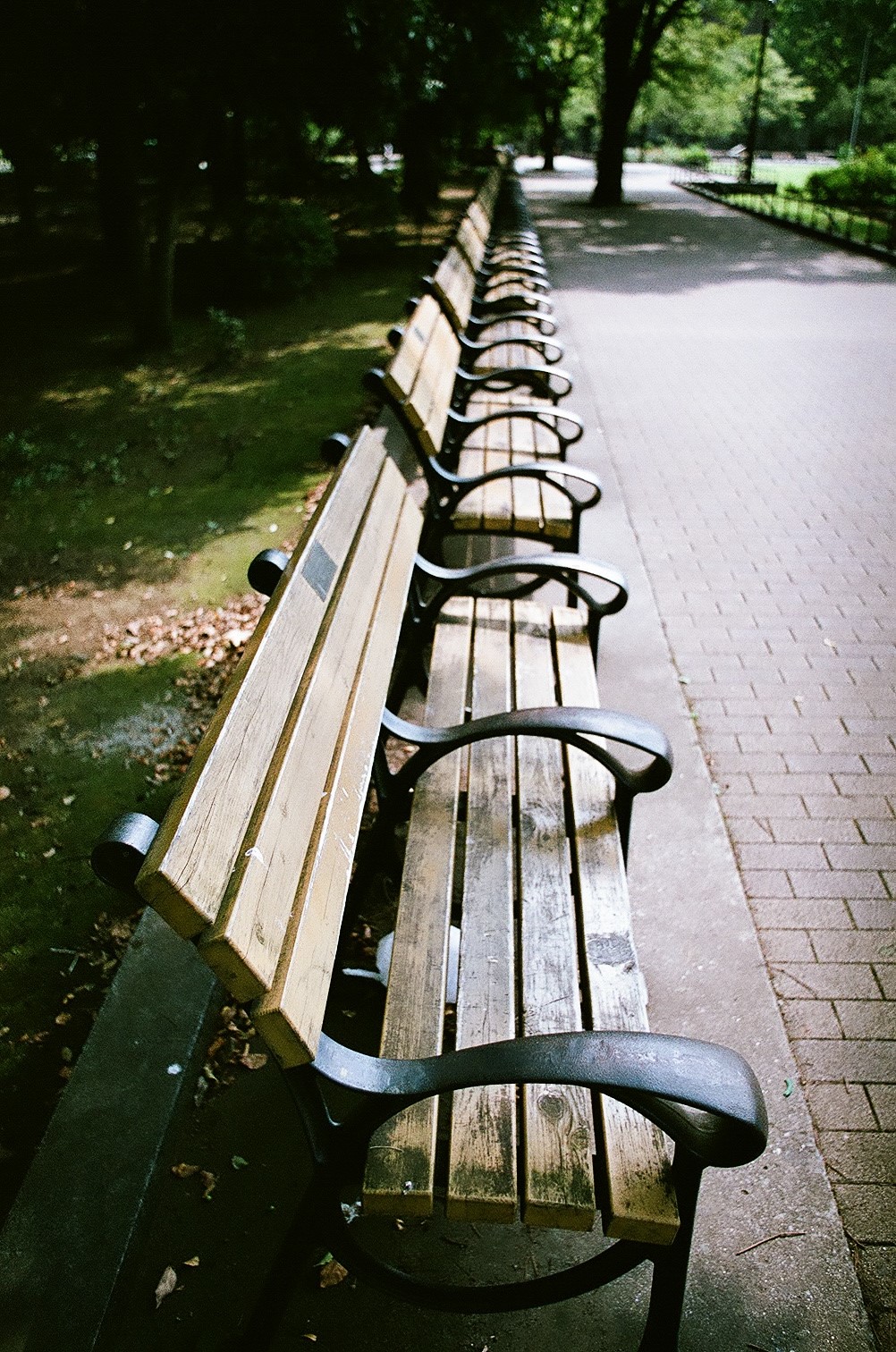This photograph captures a serene park scene featuring a long, orderly row of nine or more park benches with metal armrests and slatted wooden seats and backs. Each bench is marked with a plaque on the topmost slat, possibly for memorial purposes. The bench nearest to the camera shows signs of wear and tear, including moss growth, scratches, and chipped wood. These benches are aligned perfectly alongside a broad brick walkway that extends into the distance, indicating a well-maintained park setting. To the left, a short concrete barrier separates the benches from a lush lawn that eventually gives way to bushes around the fifth or sixth bench. The right side of the image shows a shadow-dappled sidewalk with trees periodically growing from its midst, suggesting a fall season with leaves scattered about. The overall ambiance is peaceful, enhanced by the apparent nice weather and the abundance of greenery and tree shadows.